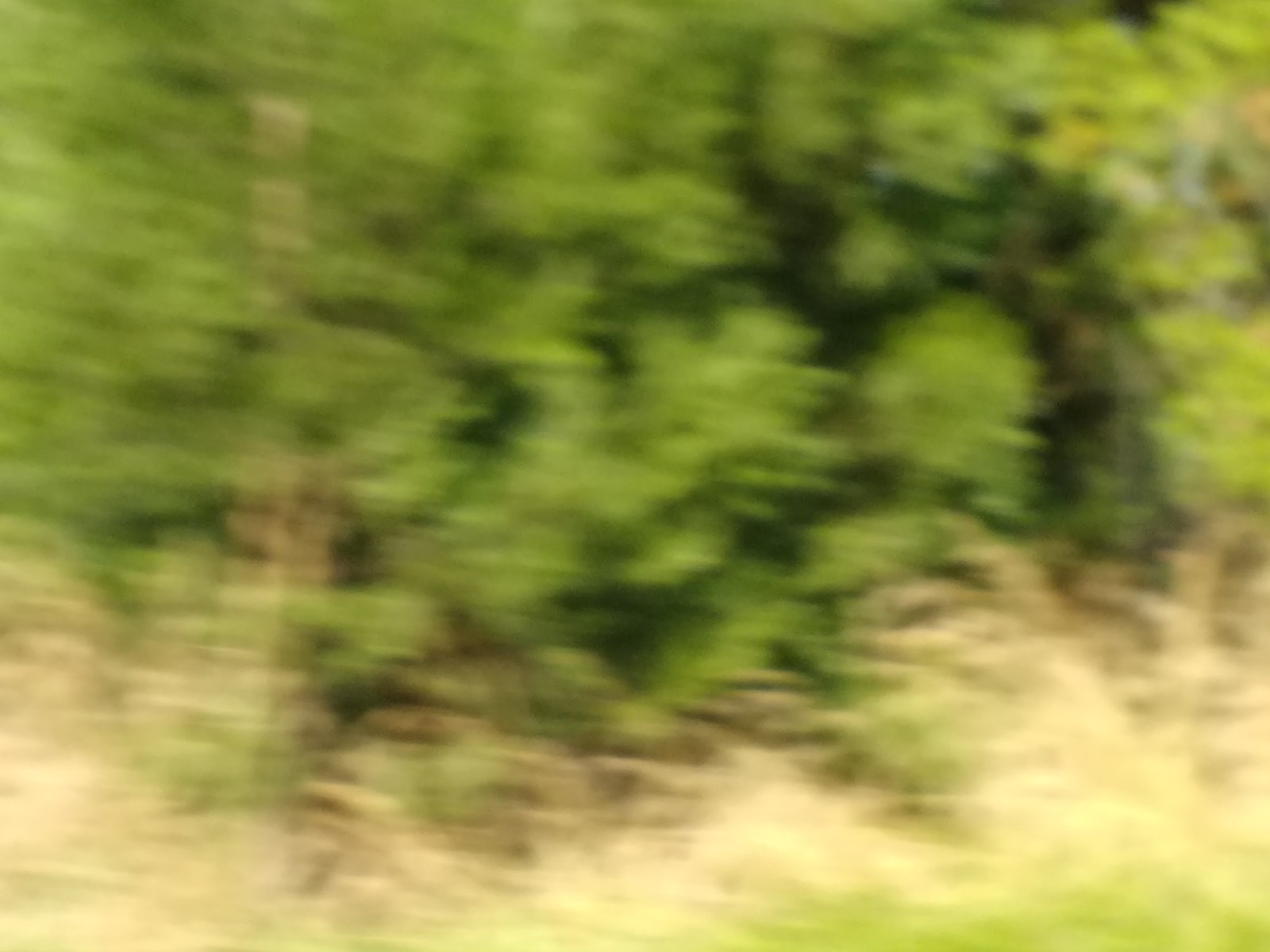A highly blurred aerial photograph captures a terrain that is difficult to distinguish. The image presents a mix of green surfaces, either grass or tree canopies, sporadically interrupted by patches of sandy ground. The sandy areas do not form straight lines but rather irregular shapes that weave through the greenery, possibly indicating a natural path or border. On the right-hand side of the photo, dark shadows create a stark contrast, hinting at the presence of trees. The overall lack of focus makes it challenging to confirm the exact landscape, but the shadows suggest a dense cluster of vegetation.